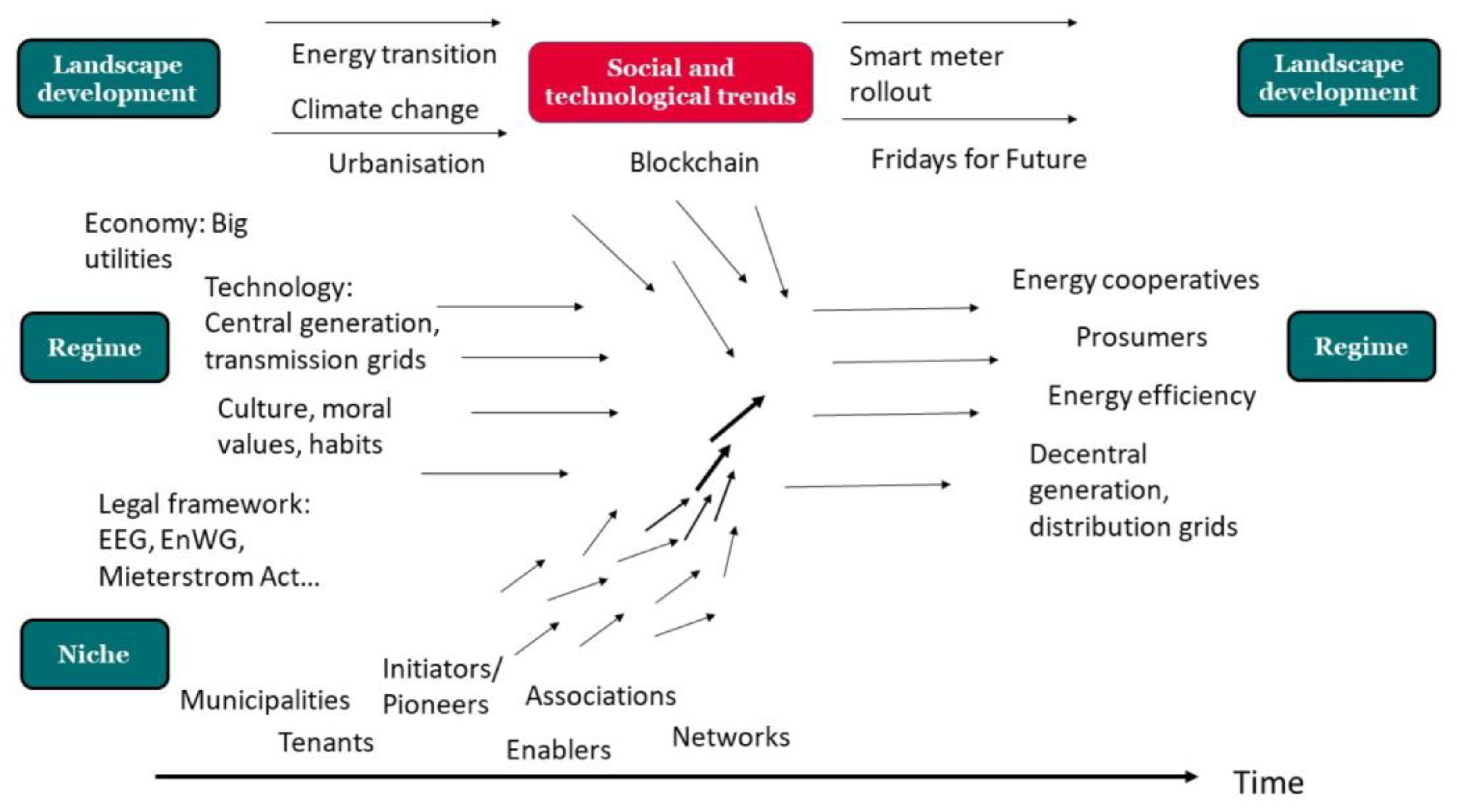The image is a detailed diagram with a white background, typically found in educational materials such as books or magazines, illustrating the concept of landscape development. In the upper left, there is a green box with a black border labeled "Landscape Development." Alongside this box, key themes are noted, including "Energy Transition," "Climate Change," and "Urbanization," with arrows pointing towards the right. 

Below this, a red rectangle with white lettering is labeled "Social and Technological Trends." This section highlights various socio-technological factors such as "Energy Transition," "Climate Change," "Urbanization," "Big Utilities," "Technology," "Central Generation," "Transmission Grids," "Legal Framework," "EEG," "ENWG," "Meaderstrom Act," and influences like "Blockchain," "Smart Meter Rollout," and "Fridays for Future."

Further down on the left side, there are two additional green boxes. The middle box, labeled "Regime," and the bottom box, labeled "Niche," contain related terms, with "Regime" associated with "Economy," "Big Utilities," and "Niche" linked to entities like "Municipalities," "Tenants," "Initiators," "Pioneers," "Associations," "Enablers," and "Networks."

Various arrows interconnect these elements, demonstrating the relationships and interactions within the broader context of social and technological change. This comprehensive diagram effectively maps out the components and dynamics of landscape development.